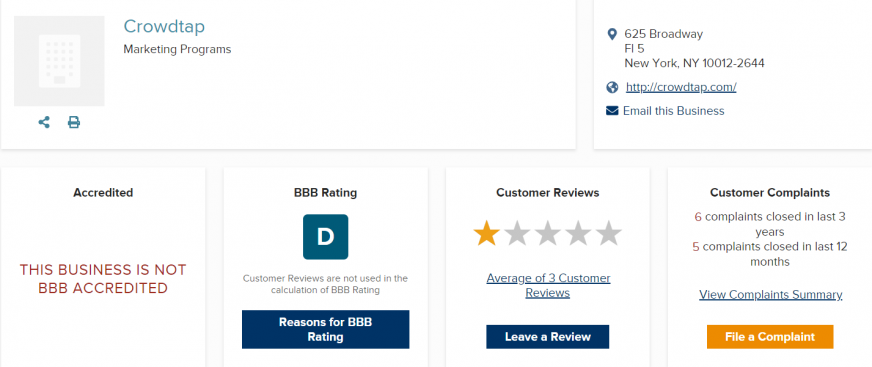**Image Caption: Detailed Review of CrowdTap Marketing Programs on Better Business Bureau**

This screenshot captures the Better Business Bureau (BBB) profile for CrowdTap Marketing Programs. In the upper left corner, the page title "CrowdTap Marketing Programs" is prominently displayed, accompanied by a barely visible, slightly discolored small square logo. On the upper right, there is a map icon next to the address "625 Broadway, 5th Floor, New York, New York," followed by the zip code. Below the address, a globe icon links to the CrowdTap website (CrowdTap.com), and an envelope icon indicates options for contacting the business. A thin line separates this section from the rest of the page.

The profile is divided into four equally spaced categories: Accreditation, BBB Rating, Customer Reviews, and Customer Complaints, suggesting it is an overview on the BBB website. In the Accreditation section, the text states that CrowdTap is not accredited. The BBB Rating section reveals a dismal "D" rating. 

Customer Reviews indicate an average of 1 star out of 5 based on three reviews, with a blue button available for reading the reasons behind this rating. Additionally, there is an option to leave a review through another blue button. The Customer Complaints section notes that six complaints have been closed in the past three years, and five complaints have been resolved in the past twelve months. A text link allows viewers to "View the complaint summary," and an orange button invites users to "File a complaint."

Overall, the customer feedback for CrowdTap is overwhelmingly negative, captured at a glance through the poor rating and reviews.